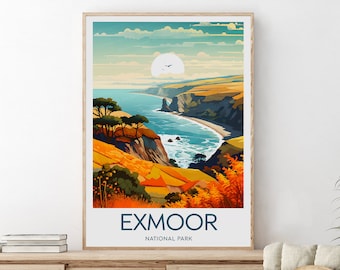The advertisement features a full-color photograph showcasing a detailed, bright, and colorful poster for Exmoor National Park. The setting is a white room with the poster leaning against a light-colored wooden table. To the left of the table, there is a stack of three closed books with their spines facing away, revealing the pages. On the bottom right, cushions or pillows are visible along with some leafy plant elements.

The poster, which appears to have a thin oak-style frame, depicts a vivid, digitally illustrated vector scene of Exmoor National Park. The main image on the poster shows striking orangey seaside cliffs lined with green trees, a beach coastline, and a serene body of blue water draped in teal clouds. A large sun sets in the background, casting warm hues across the scene. Below the image, "Exmoor National Park" is clearly printed on the white background of the poster.